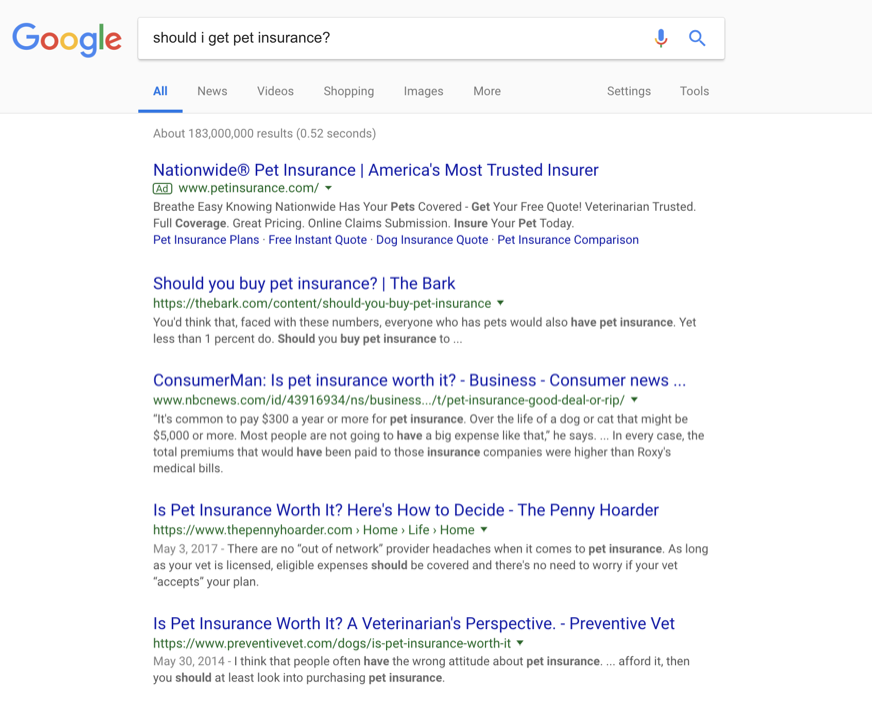The screenshot captures a Google search results page with the query "Should I get pet insurance?" entered into the search bar. Below the search bar, there are navigation tabs: "All" (highlighted in blue, indicating it's the active tab), followed by "News," "Videos," "Shopping," "Images," and "More." On the far right of the screen, options for "Settings" and "Tools" are visible. The search has yielded approximately 183 million results in 0.52 seconds.

The initial search result is an advertisement from petinsurance.com, titled "Nationwide Pet Insurance, America's Most Trusted Insurer." The subsequent organic result is from thebark.com, titled "Should You Buy Pet Insurance? - The Bark." The third result, from NBC News, is titled "Consumer Man: Is Pet Insurance Worth It?" The fourth result, found on thepennyhoarder.com, is titled "Is Pet Insurance Worth It? Here's How to Decide." The fifth and final visible result is from preventivevet.com, titled "Is Pet Insurance Worth It? A Veterinarian's Perspective," found under their dog section.

The background of the page is white, with titles of the websites in blue and the URLs in green.